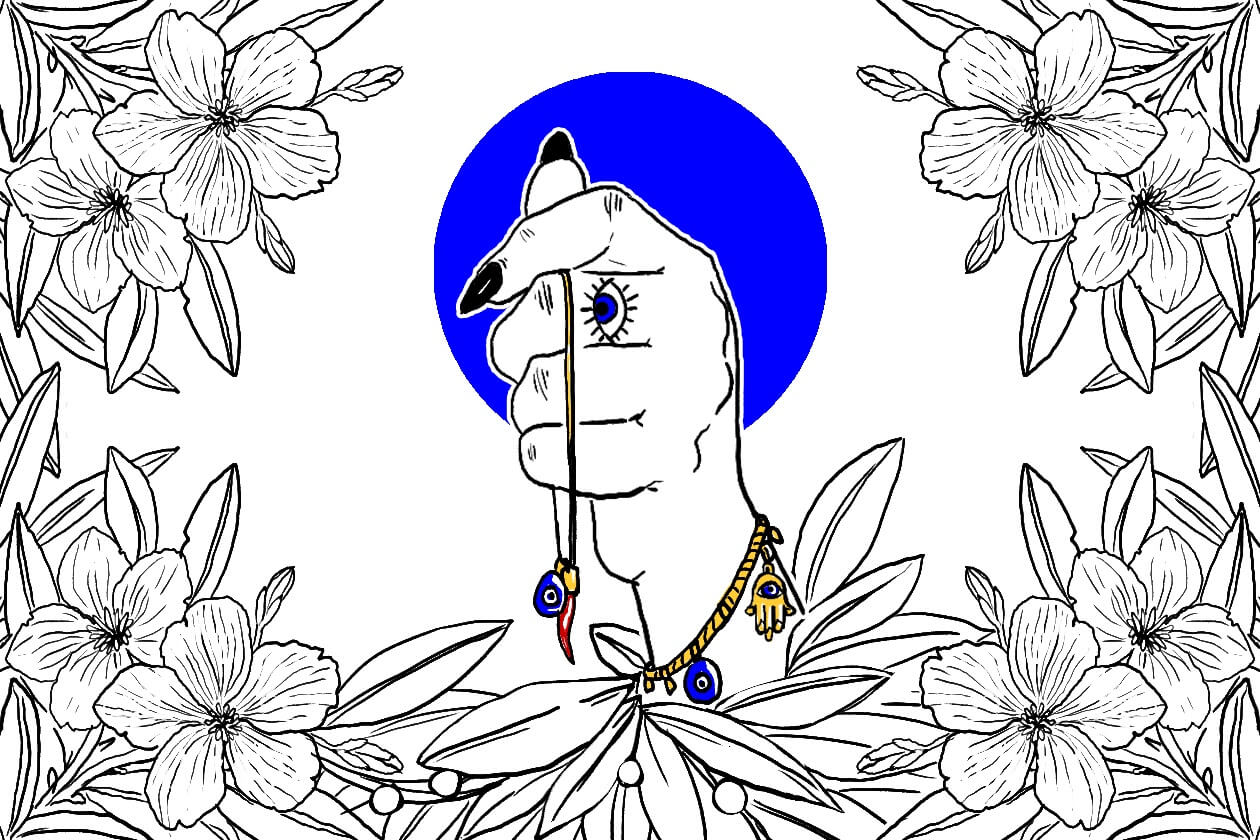This black and white line art illustration, accented with spot color, is presented in a landscape orientation and features a detailed floral motif bordering the left, right, and bottom sides. The border is composed of intricate outlines of various flowers, including hibiscuses and dogwood blossoms, interspersed with leaves. At the center of the composition is a prominent blue circle, behind which a woman's hand is depicted emerging. The hand, folded inward towards the palm, is adorned with a long black nail on the index finger and thumb. Notably, this hand wears a striking ring on the middle finger, showcasing a sideways eye with a blue iris and long black eyelashes. Draped over the folded fingers is a chain leather strap, from which dangles a colorful charm resembling a bird's head in blue, red, and yellow hues. Additionally, the wrist is accessorized with a gold-colored bracelet featuring two distinct charms: a Hindu hand symbol and a round blue disc. This illustration melds detailed line art with selective use of color to create a captivating visual experience.